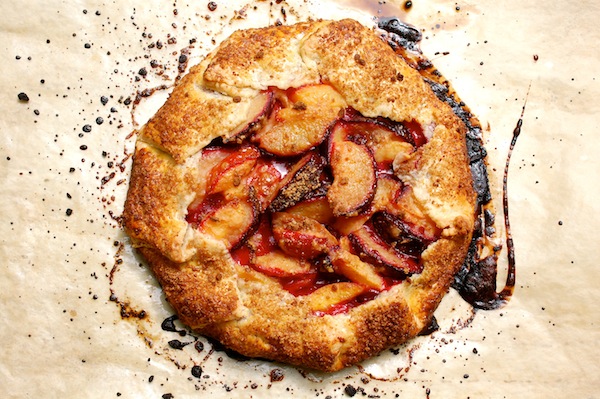The image depicts a delicious-looking baked pastry, reminiscent of a galette, featuring a golden-brown, slightly burnt crust with speckled burnt areas, particularly on the right side. Nestled inside the pastry are slices of fruit, likely a mix of apples, peaches, or nectarines, identifiable by their yellowish-orange flesh and red skins. Surrounding the pastry are small black dots, possibly drips of jelly, emphasizing the fruit filling. The pastry sits on a tan or beige wax paper, which has also browned, presumably from being baked in the oven. The whole scene is set against an off-white background.